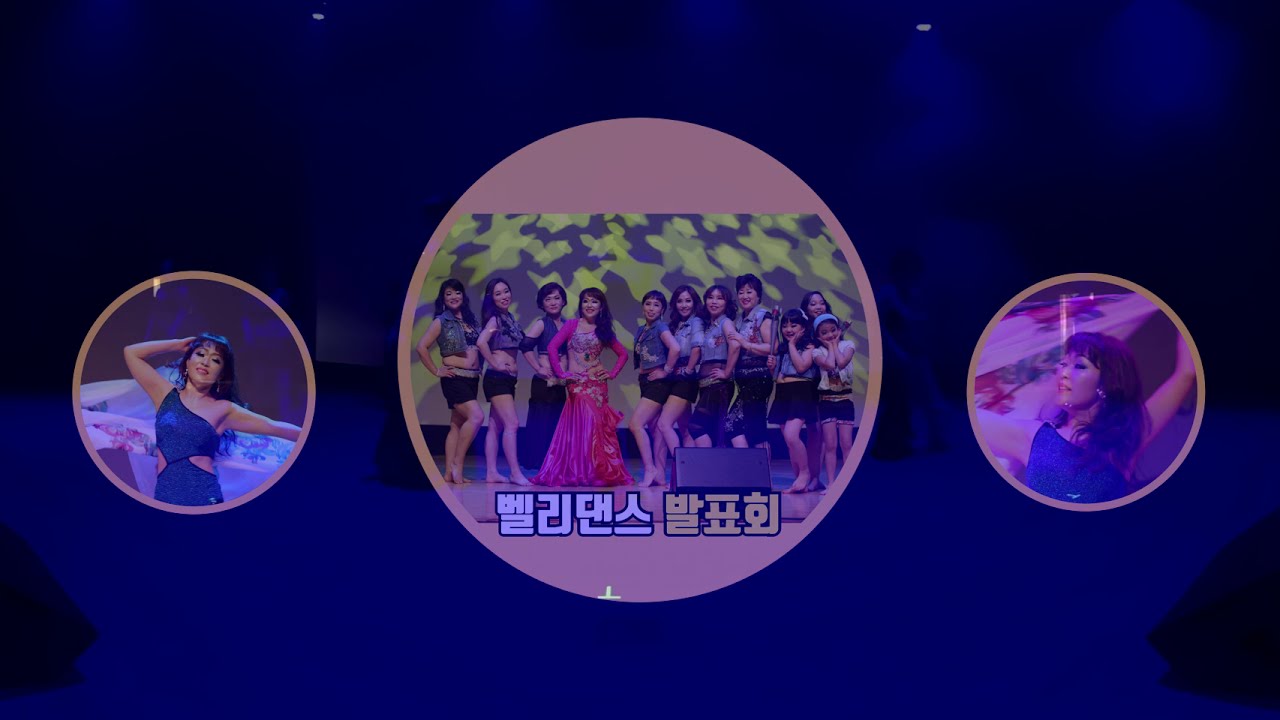The composition showcases a performance or competition scene centered around young women posing onstage. The image is divided into three circular photographs with beige borders, set against a blue background that features a blurred-out version of the main image. The primary circular photograph in the middle displays approximately eleven young women, dressed in performance outfits, standing in front of a green patterned wall with Asian script below them, possibly Korean or another Asian language. Flanking this main photo are two smaller circles highlighting individual women in blue dresses with cutout details near the waist, each striking a distinct pose. The blue background of the entire image, interspersed with light and dark blue tones and spotlights, evokes a stage-like atmosphere.